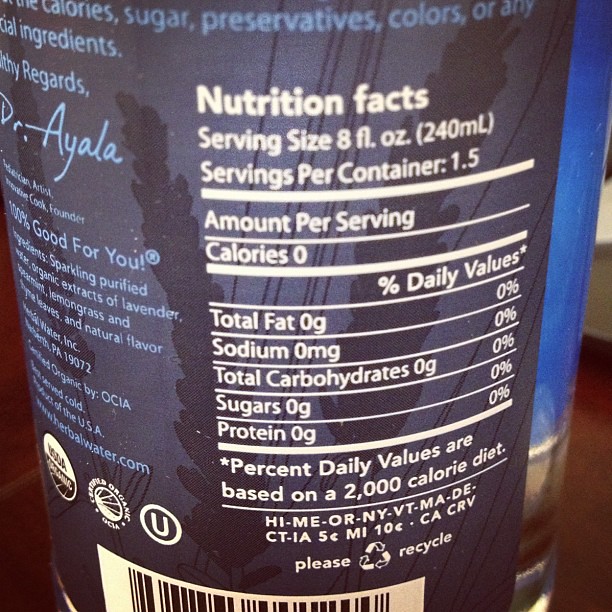The photo showcases the nutritional facts on the back of a blue canned beverage. Dominating the scene is a dark blue rectangle highlighting key nutritional data: serving size of 8 fluid ounces, 1.5 servings per container, and zero values for calories, fat, sodium, carbs, sugars, and protein. In the lower section, various deposits (5 cent and 10 cent) and a "please recycle" icon are visible, along with a partial view of the barcode. On the left, there is some information about the drink's beneficial attributes, signed by Dr. Ayala. The ingredients listed include sparkling purified water, organic extracts of lavender, spearmint, and lemongrass, with natural flavorings. Certified organic and PARV symbols, indicating kosher status, are also featured.